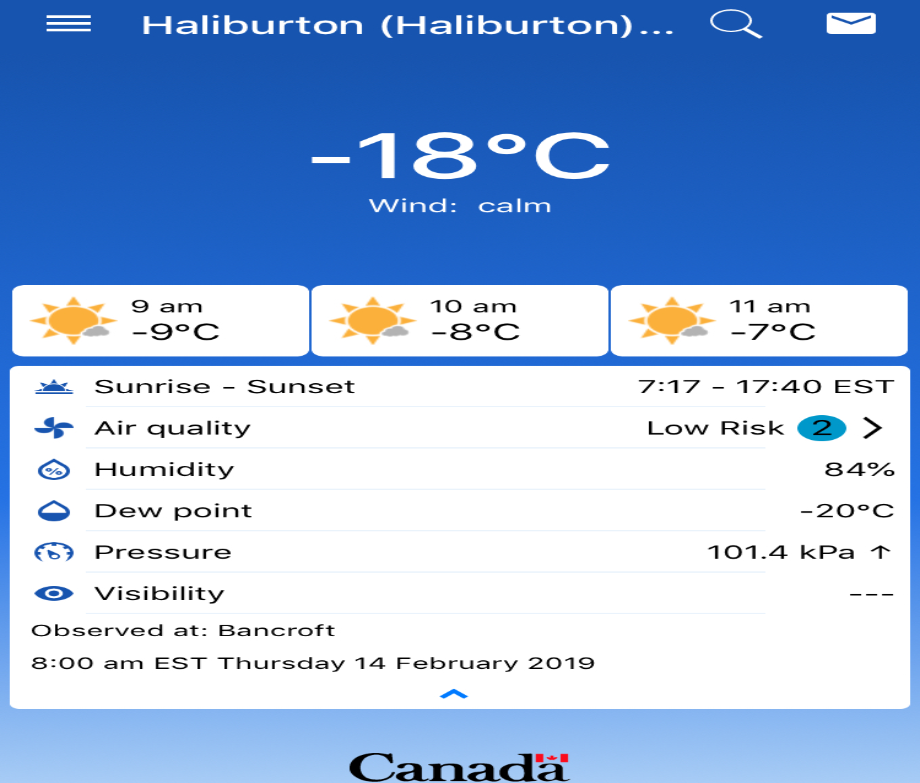This screenshot showcases a weather application interface with a navy blue to light blue gradient background. At the top, there's a context menu on the upper left-hand side, featuring three lines next to the word "Halliburton," followed by "Halliburton" in brackets. Adjacent to this are three dots for additional options, a search function, and an email icon.

Central to the display is the current weather condition, stating -18°C with calm winds as of 9 a.m. Below this, a three-hour forecast is provided:
- 9 a.m.: Partly cloudy, -9°C
- 10 a.m.: Partly cloudy, -8°C
- 11 a.m.: Partly cloudy, -7°C

Further details include the sunrise and sunset times at 7:17 a.m. and 5:40 p.m. Eastern Time. The air quality is rated low risk with a marking of 2, circled in blue. Humidity is high at 84%, with a dew point of -20°C. Atmospheric pressure is listed as 101.4 kPa and is rising, whereas visibility is represented by a series of dots and dashes. 

The observation was noted in Bancroft at 8 a.m. Eastern on Thursday, February 14, 2019. At the bottom of the screen, the word "Canada" is displayed in black, accompanied by a small Canadian flag over the letter "A."

Icons supplement the text, including a blue sunrise, a windmill, two water droplets (one with a percentage and one half-full), a pressure gauge, and a blue eye symbolizing visibility. This detailed overview illustrates the design and information provided by this weather app.